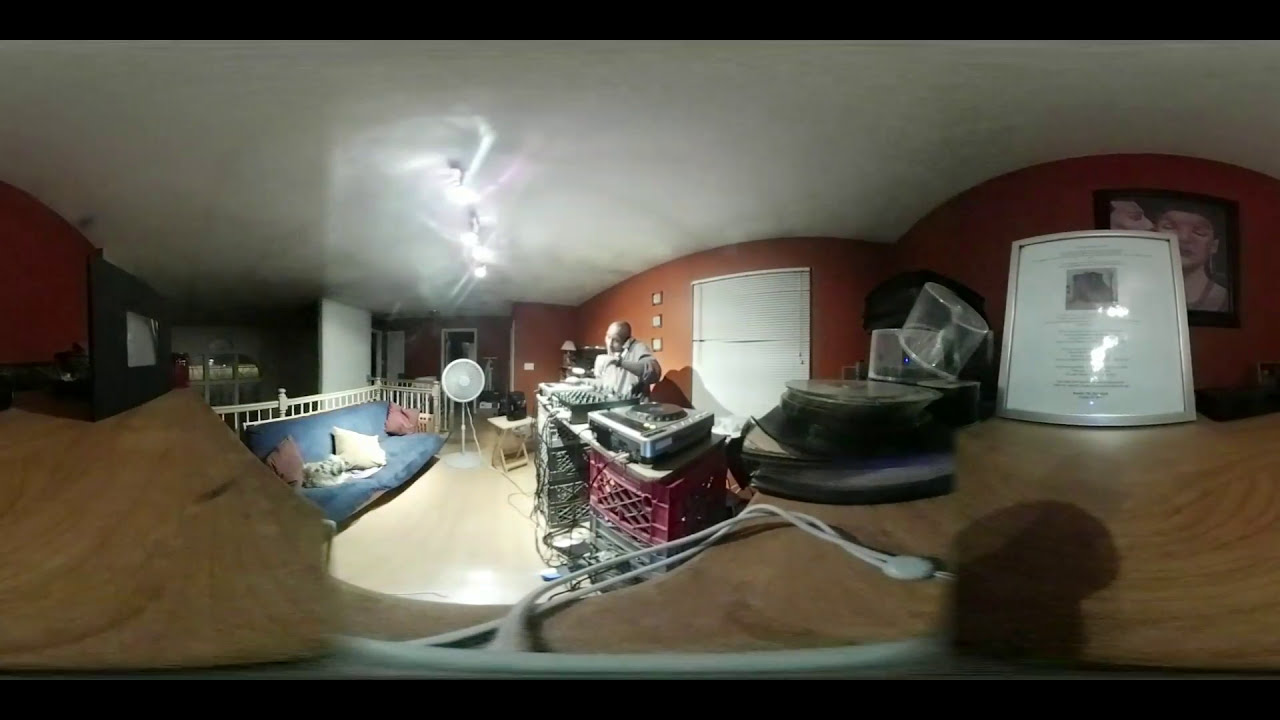The image depicts a spacious living area, possibly a basement, with terracotta brown walls that appear curved due to lens distortion. On the left side, there's a blue futon adorned with pink and white pillows. Central to the scene stands a young man practicing his DJ skills, engrossed in his setup, which consists of a turntable and a mixer housed upon a makeshift table formed by a large board balanced on gray and pink plastic crates. He’s positioned in front of a window with white blinds. The photograph seems to have been taken from an elevated vantage point, possibly a wooden shelf, which is partially visible in the foreground along with a white cord. On the right side of the room, there is a framed photo depicting a man and a woman, and adjacent to it, another framed certificate or diploma is visible, albeit partially obscured by reflective glare. Additional details include a standing fan to the left and a marble countertop that suggests the room is part of a larger living space, possibly the second story as hinted by elusive handrails that could belong to a staircase.